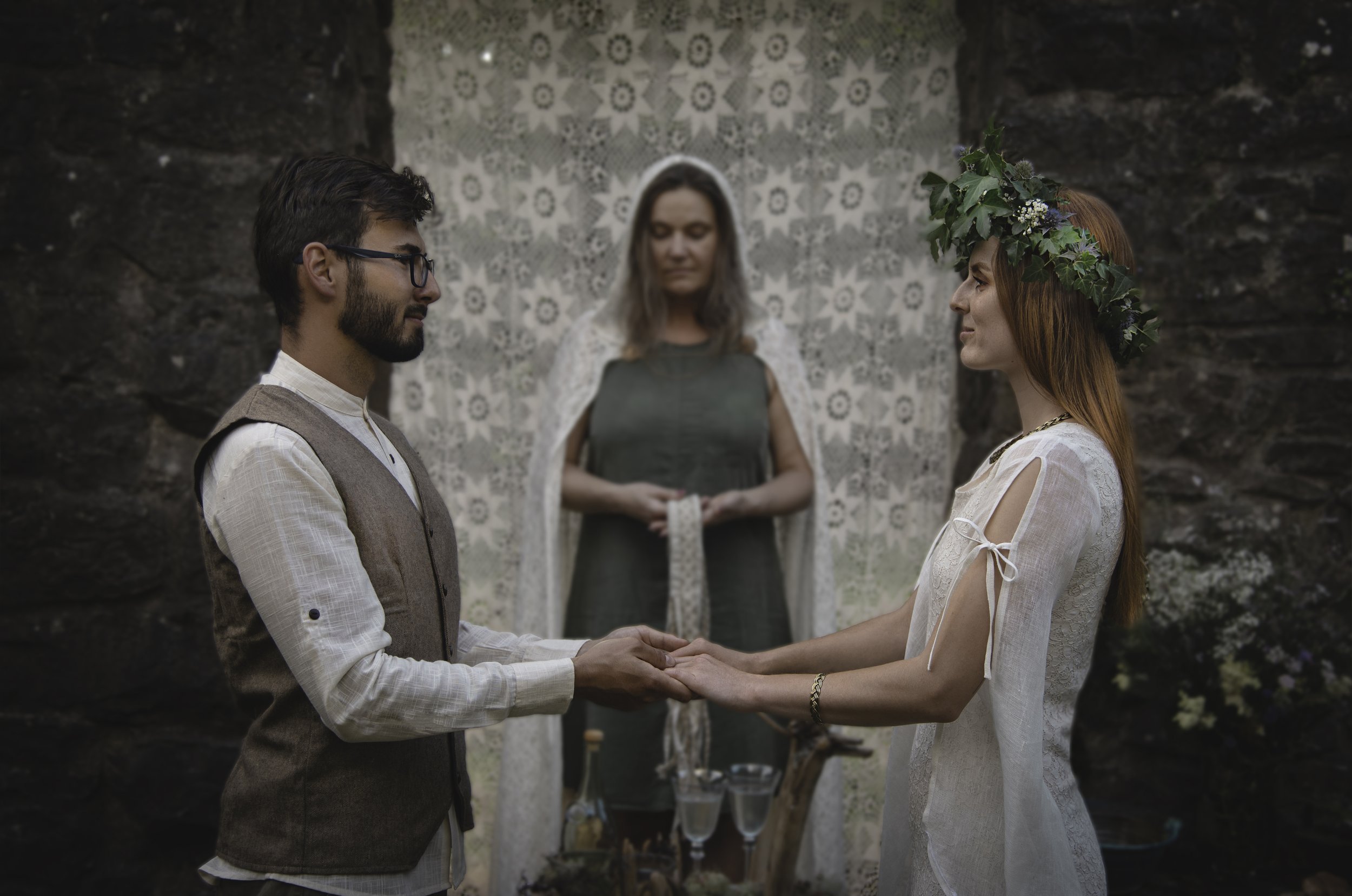In this photograph, a solemn Celtic-style wedding is depicted against a dark stone wall adorned by a white and grey patterned tapestry hanging down its center. In the background stands an officiant, draped in a simple grey dress and a white cloak with a hood, her long brownish-grey hair cascading as she looks downwards. Her figure appears slightly blurred. Beside her are two glass goblets containing a clear liquid and a corked glass bottle. 

In the foreground, the bride and groom stand facing each other, their hands joined. The groom is attired in a white linen shirt beneath a grey vest, sporting short dark hair, a dark beard, and black-framed glasses. The bride wears a thin, gauzy white dress exposing her arms, accentuated by a bow on the exposed arm and a silver band on her forearm. Her long red hair is adorned by a green and purple wreath. The scene captures the intimate moment they share, suggesting the commencement of a new journey together.